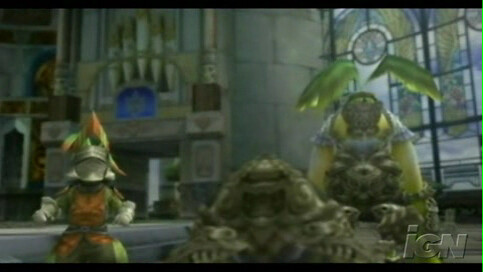This screenshot from a video game features a scene set inside a dark and shadowy church, characterized by its cartoonish design. In the background on the right side, there are intricate stained glass windows, while the left side reveals a church organ or a similar structure against a cement or cinder block wall. Three distinct characters, all clad in armor, are positioned prominently within the church. 

The character on the left is dressed in knight's armor and sports a red shirt underneath, accented with a red and green flag protruding from the top of their helmet. The middle character appears as a short, blob-like figure, enveloped entirely in gray armor. The character on the right stands taller than the rest, adorned in yellow attire with gold armor and topped with two green flags. The contrasting heights and colorful armor of the characters add a lively touch to the otherwise dim and moody ambiance of the church setting.